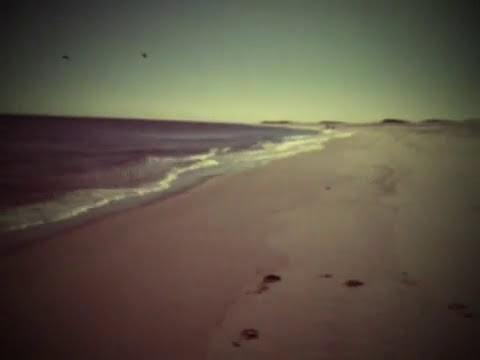This image captures a serene beach scene characterized by its untouched expanses of sand and tranquil waters meeting at the shoreline. On the right side of the image, an extensive stretch of slightly worn sand extends, with occasional footprints hinting at limited human activity. To the left, the clear blue waves of the ocean gently crash against the shore. Above, the sky is a vivid blue, unmarred by clouds and inhabited by two black birds in flight. In the far distance on the upper right, a land mass is faintly visible, resembling mountainous terrain or large hills. The colors in the image span shades of blue, black, white, green, orange, tan, light brown, dark brown, and a sepia-like filter that gives it a slightly old photograph appearance. The scene overall evokes a calm, untouched natural beauty, emphasizing the solitary, undisturbed nature of the beach set under the clear midday sky.